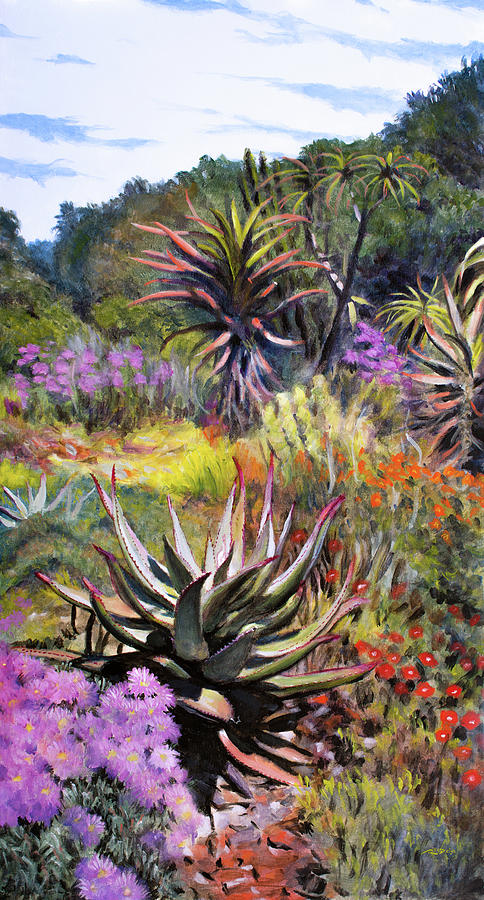This vibrant rectangular painting, likely created using either watercolor or oil pastel, presents a surreal and lush tropical landscape. Dominating the composition is a lively assortment of exotic and desert vegetation, densely packed in the foreground. The scene features colorful desert and tropical plants in hues of violet, green, and orange, including several spiky cacti or succulents with green and red-tipped leaves. Scattered among these are vividly colored flowers—red, orange, and yellow—alongside purple flower bushes, enhancing the vibrant palette.

The middle ground transitions into taller, thick green trees that evoke a more tropical setting, suggesting a lush forest or hillside. These trees extend up a slope or hill, contributing to the sense of depth and height in the image. Above, the sky is mostly cloudy with slivers of bright blue peeking through, illuminating the scene with natural light. The overall effect is a bright and dynamic representation of a surreal, tropical paradise, teeming with diverse and colorful flora.